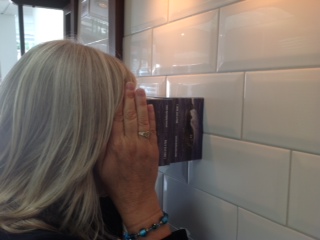In a perplexing scene, a middle-aged woman with blonde or partially gray hair stands in a tiled room, potentially a bathroom, with a window or glass door behind her letting in daylight. She is facing and appears to be intently looking into a small box pressed against the white tiled wall. Her right hand, adorned with a gold ring on her ring finger and a blue gemstone bracelet on her wrist, is raised beside her head, obscuring her face from view. Her attire includes a dark-colored sleeve, hinting at a jacket or top. The image's composition and the woman's actions give it an odd, mysterious quality.